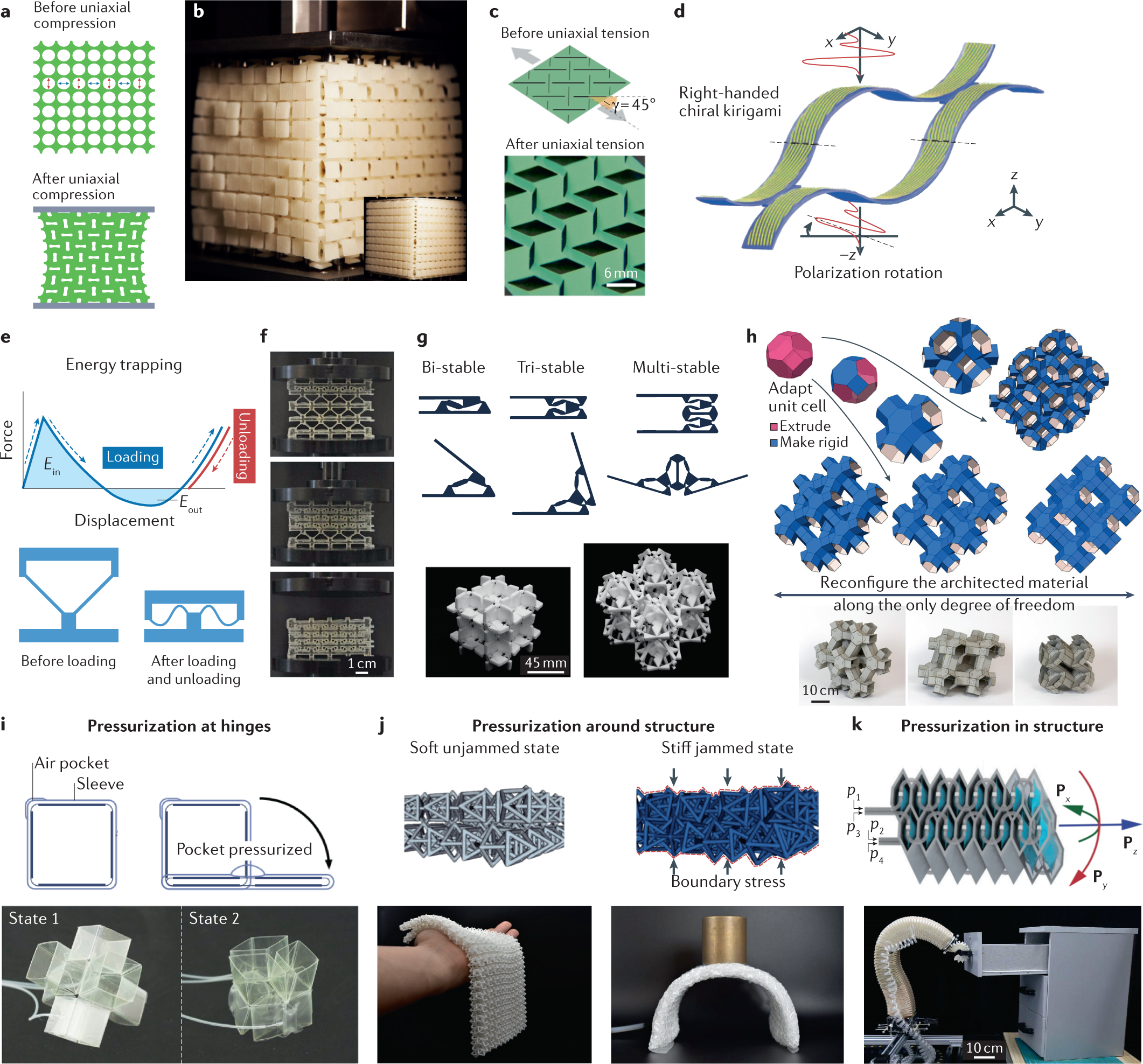This detailed image illustrates the various properties and transformations of a flexible, architected material through a series of labeled sections from A to J, each visually and descriptively presented. In the upper left, section A includes two green grid-like images of the material under uniaxial compression, showing states before and after compression with visual deformation at the center. Adjacent to it, sections B and C continue with images depicting the material under uniaxial tension, transitioning from a relaxed state to a 3-dimensional view. Section D is characterized as "Right-handed chiral kirigami," displaying two wavy strips of the material. 

The middle row begins with section E, which discusses energy trapping, showing a parabolic graph of force versus displacement during loading and unloading. Section F presents three images of the material, though their small size makes details indiscernible. In section G, the material is demonstrated in bistable, tristable, and multistable states, with corresponding images of a cuboid shape and clustered spheres. Section H shows adaptive capabilities, with a sequence of operations: adapting unit cells, extruding, and making the material rigid, supplemented by different shape displays.

At the bottom, section I addresses pressurization at hinges, showing air pockets and different material states labeled as "pressurized pockets," accompanied by images denoting two different structural states. Section J focuses on the impact of pressurization around the material structure, contrasting a "soft unjammed state" resting in a person's hand with a "stiff jammed state" supporting a copper cylinder in an arch shape.

Every detail, step, and transformation is comprehensively laid out using a combination of photographs, diagrams, and graphs on a white background, with color-coded sections in blue, green, black, and red, elucidating the material's versatility and advanced engineering applications.